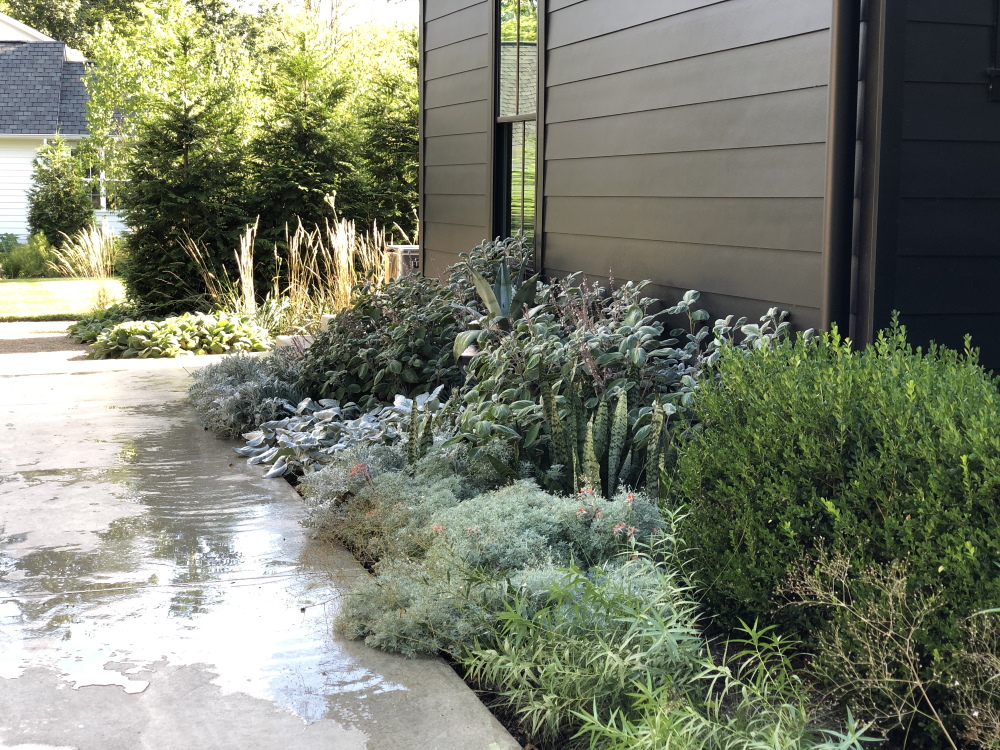This photograph captures the side of a dark brown paneled house, likely located in a suburban area. The visible portion of the house occupies the upper right quadrant of the image and features a single portrait-oriented rectangular window, subdivided into three smaller panes. Adjacent to the house is a lush garden filled with a variety of healthy, green plants and shrubs, which exhibit different textures and shades of green but no visible flowers. The garden extends to a light concrete driveway, which appears slightly wet, suggesting recent rainfall or watering. Moving further to the background, a more softly focused scene reveals an assortment of trees and the roof of a distant white house with a black roof. The entire scene is bathed in sunlight, indicating a bright, clear day.